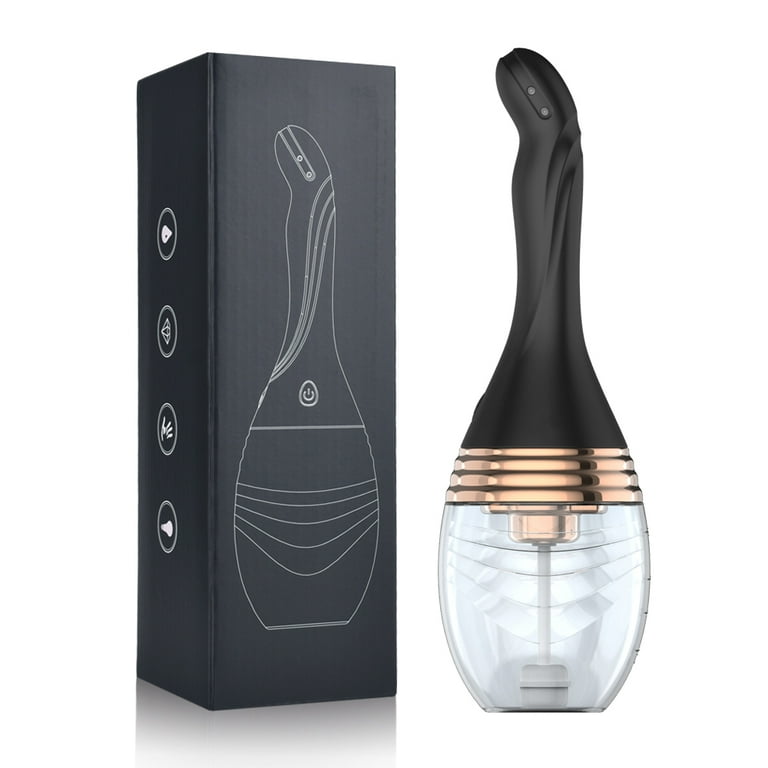The photograph features a unique and intriguing device with a design reminiscent of a perfume bottle or decanter, shaped similarly to a bowling pin. The device has a clear glass-rounded base and an elongated, black plastic neck with ridges at the top, connected by a brass-colored metallic band. The upper portion ends in a handle with a pointed tip that extends to the side. Inside the device, there is a clear portion of white plastic dipping into the middle of the glass. 

To the left of the device is a sleek, black box that appears to be the packaging for this product. The box's surface facing the viewer has a line drawing of the device, displaying four circles likely indicating the product's features. There is also an illustration of a power button, which is not visible on the physical device in the photograph. The overall image provides a detailed visual description of the product and its packaging, emphasizing the contrast between the rounded, clear base and the ribbed black neck, enhanced by the metallic accent.